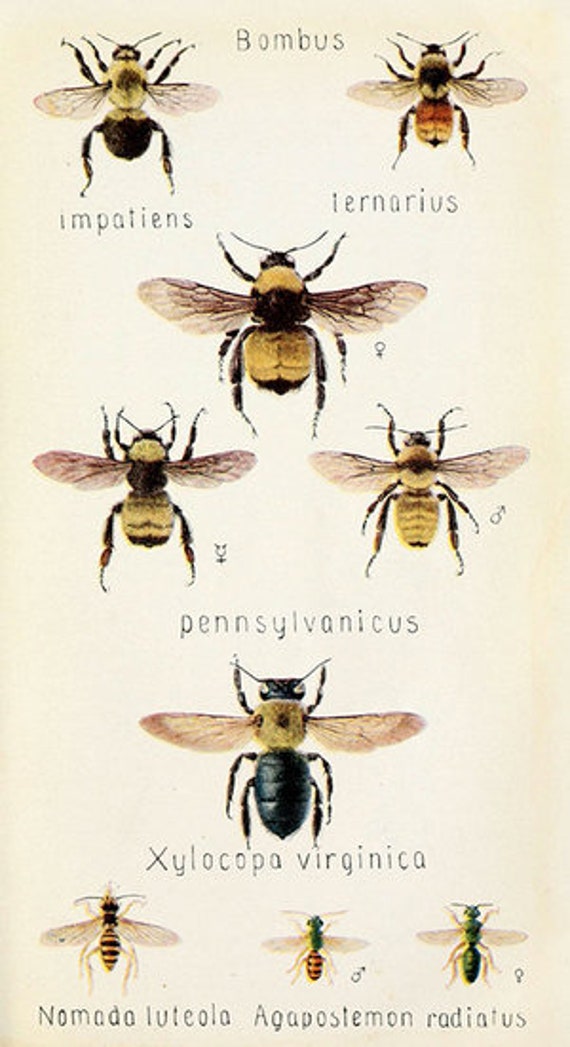This is a detailed chart of various bee species, set against a white background with a gradient of yellow and tan shading around the edges. Prominently displayed in the center is the word "Bombus" in gray lettering.

In the upper left corner, there is an illustration of a bee with a distinctive black abdomen, a yellow body adorned with a brown spot in the middle of its back, and translucent wings. Just to the right, another bee is depicted with a striking red and yellow tail. Its body is predominantly black, highlighted with white around the edges. 

Directly below these, at the center of the chart, is a bee whose abdomen is yellow with a hint of black at the tip. It features a black circle on its back and a yellow front portion near its head. 

Below this bee, to the left, is one that has a light yellow abdomen accented with horizontal black lines across it and a yellow body. To its right, another bee showcases an abdomen that's yellow transitioning to beige at the top. This bee's body is white with a central brown marking.

Further down, another bee is illustrated with a black abdomen, while its upper body transitions to a pale yellow-brown color with a brown dot in the center. Below this bee, on the left, a smaller bee can be seen, featuring a yellow tail with black horizontal lines and an entirely black body. 

To the right of this smaller bee, there is one with a gold-colored abdomen and a green body, followed by yet another with both a green abdomen and body. All these bees are depicted with wings and legs, each accompanied by scientific names written underneath, though they are difficult to pronounce.